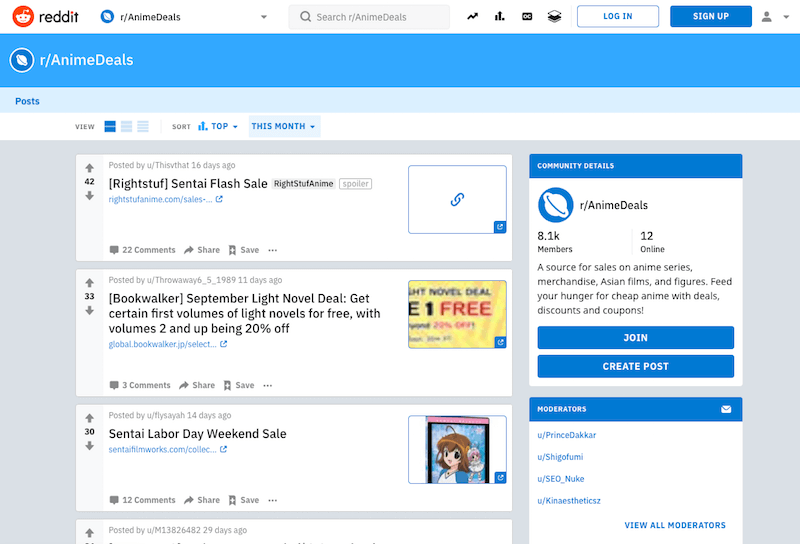The image displays a section of Reddit specifically targeted at anime deals. Starting in the top left, the Reddit logo and the word "reddit" are prominently displayed next to the iconic orange Reddit mascot. The browser tab is titled "Our Anime Deals." Adjacent to the title is a search bar, followed by a series of four or five black icons and buttons for logging in and signing up.

Beneath this header, a blue banner with white text reads "Our Anime Deals." Directly below, "Posts" is situated in the top left corner. Further down, options for viewing posts are available with three distinct viewing modes, along with sorting options labeled "Top" and "This Month."

The main content area features three highlighted deals in rectangular boxes. The first rectangle showcases a "Right Stuf (Sente) Flash Sale," accompanied by a blue website link and 22 comments. The second deal, labeled "BookWalker September Light Novel Deal," promotes certain first volumes of light novels for free, with subsequent volumes available at a 20% discount. The third rectangle advertises a "Sentai Labor Day Weekend Sale," which also includes a website link.

On the right-hand side, the "Community Details" section is visible, listing 8.1k members and 12 members currently online. This section describes the community as a source for sales on anime series, merchandise, Asian films, and figures, encouraging members to "Feed your hunger for cheap anime with deals, discounts, and coupons." Below this description are buttons to "Join" and "Create Post," followed by a list of moderators.